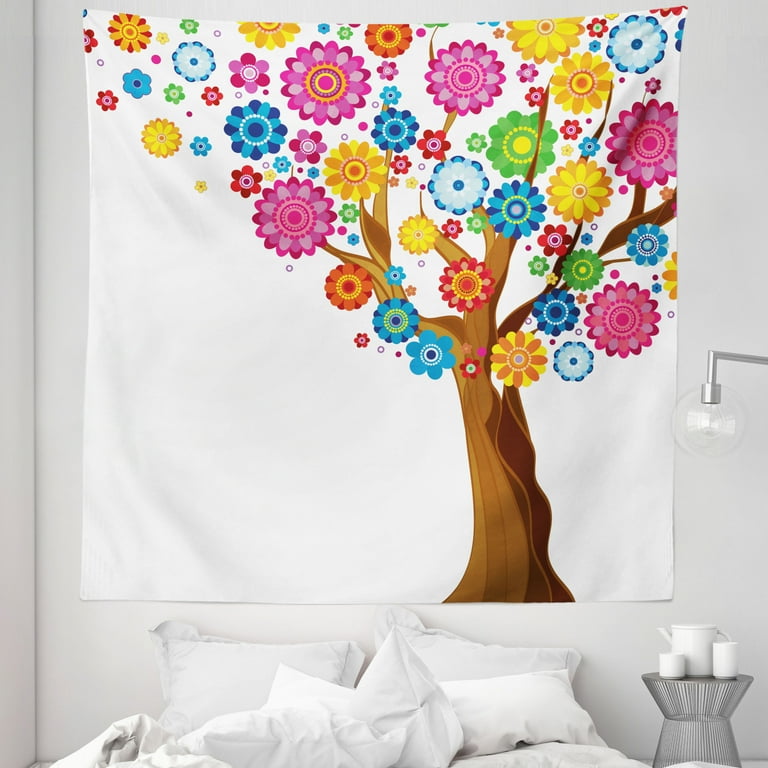The bedroom in the image features tall, medium white-gray walls, with the corner of the room visible on the left side. Against the back wall lies a bed adorned with white linens, including four scattered pillows and a crumpled comforter. Adjacent to the bed, on the right, stands a modern, hourglass-shaped nightstand made of silver wire, holding a white pitcher and two white glasses – a tall drinking glass and a shorter coffee mug. Above the nightstand, a sleek silver lamp extends from the wall at a sharp right angle, featuring a large, clear round bulb.

Dominating the space above the bed is a large white fabric tapestry. It showcases a simplified tan tree with branches extending outward. Vibrant, geometric flowers in shades of pink, blue, yellow, green, and more are scattered across the tapestry, some appearing to float away from the branches, adding a burst of color to the serene setting.